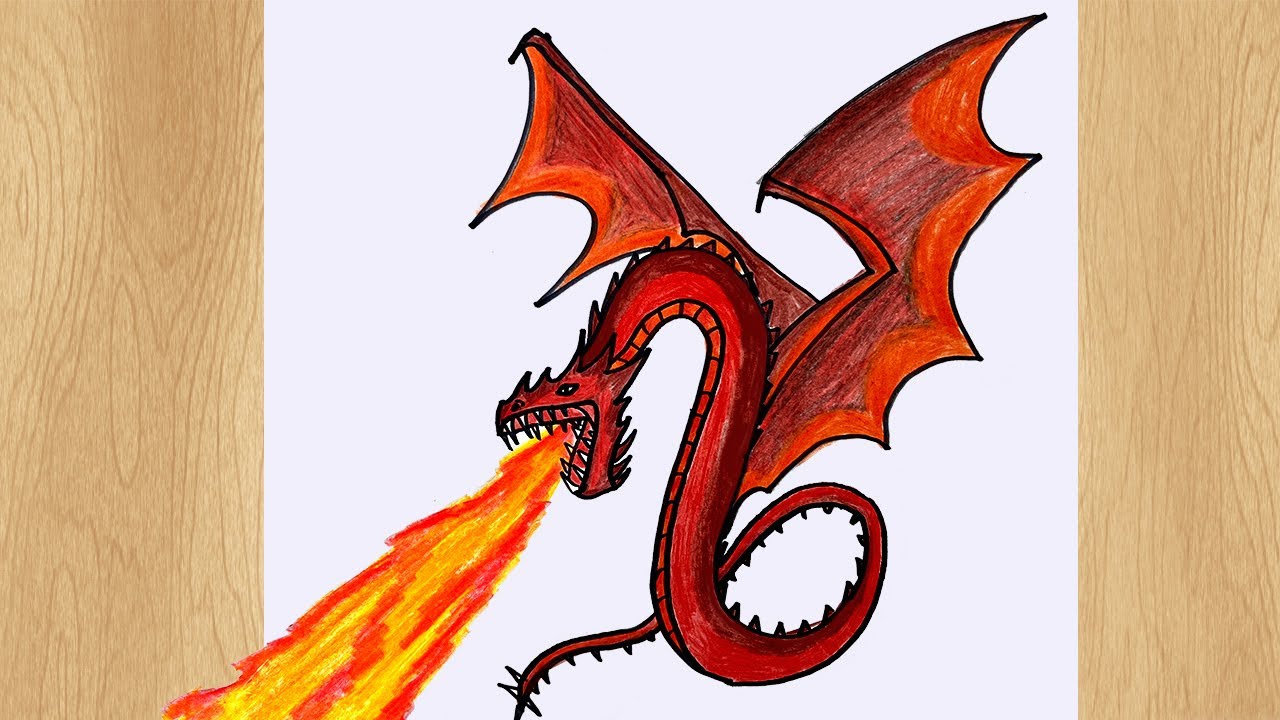This is a detailed illustration of a medium-sized, red, fire-breathing dragon, meticulously drawn with a black ink pen and colored using crayons or colored pencils. The dragon features a sinuous, snake-like body with no legs and is adorned with sharp black spikes running along its back, head, and jawline, culminating in menacing, spiked teeth. Its two wings, which are red with orange outlines, are spread wide as it hovers, blowing a fierce stream of flames that transition from dark red to yellow-orange. The vibrant fire appears to almost leap off the white sheet of paper. This paper rests on a light brown wooden surface with visible grain, adding a natural backdrop to the dynamic scene.